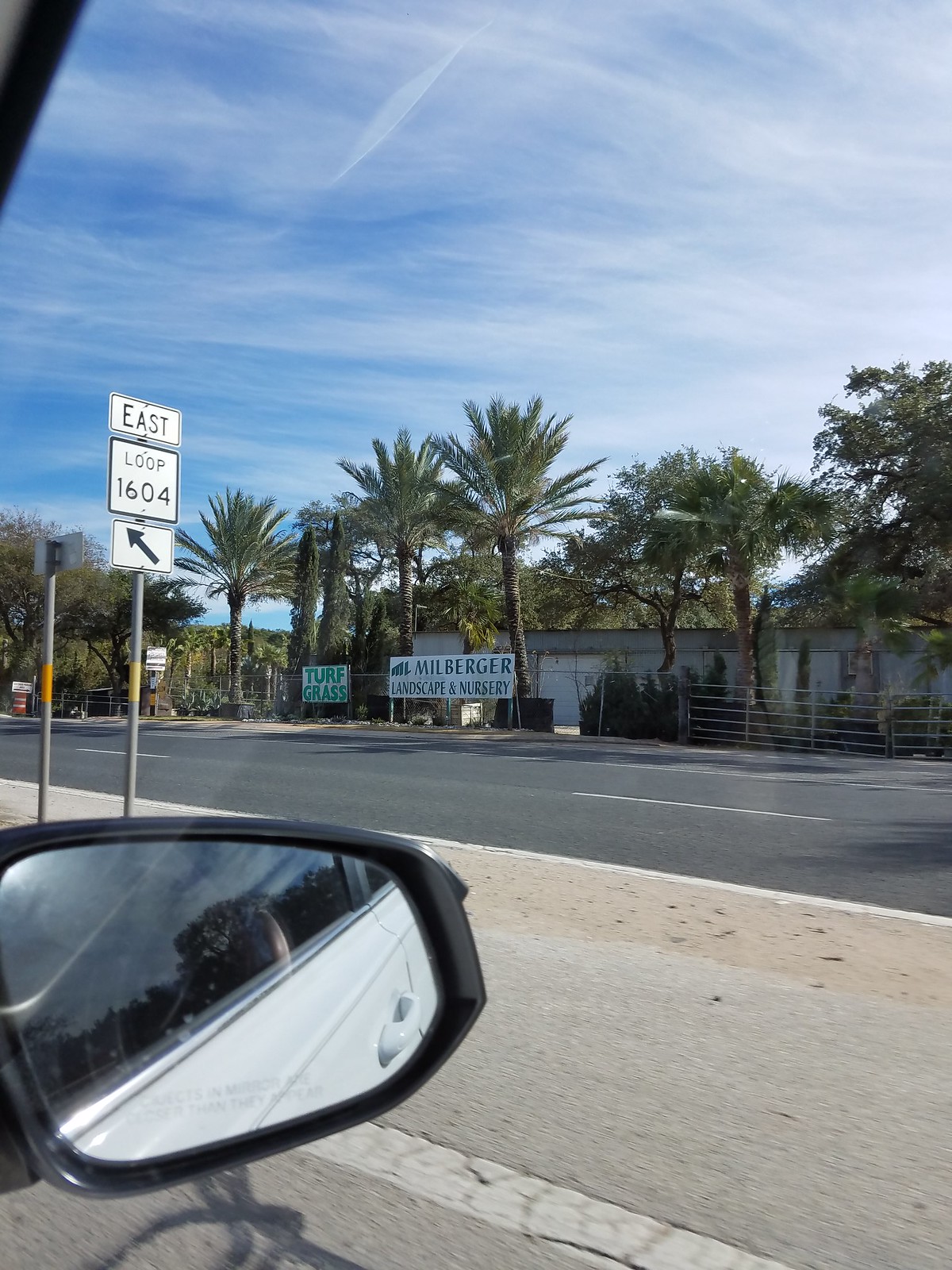A detailed view from the passenger seat of a white vehicle is captured in this image. In the bottom left corner, the car's side mirror is visible, reflecting the vehicle itself. The area visible in the mirror shows the white car’s body. In the background, the scenery is composed of several single-story buildings, alongside numerous tall and lush green palm trees and other regular trees. Adjacent to these trees, a chain-link fence runs parallel with the road, festooned with various signs, one of which reads "Caution" and another, partially obscured, reads "No Parking." Running parallel to the fence is a road extending from the right edge to the left of the image. Beside the road, there is an island or sidewalk area that features a street sign positioned towards the top left corner of the image.